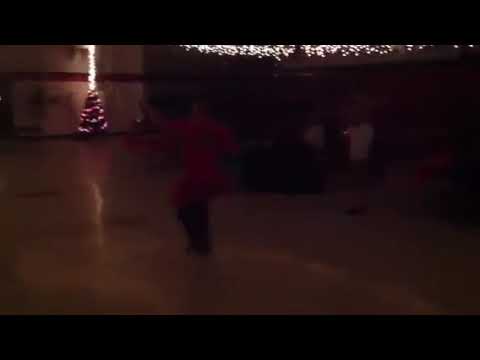The image is a very dark and blurry photograph, possibly taken at night, depicting a festive scene. In the center, a woman in a red dress appears to be the focal point, possibly dancing. To her left, there is a small Christmas tree adorned with lights, perched on a shelf. White Christmas lights are seen hanging above, and more lights extend to the right of the woman. In the background, partially visible silhouettes of two individuals in white shirts, one of whom may be wearing tan pants, can be discerned. The floor seems white, possibly covered in snow or reflecting the ambient lights. The photo has a black frame at the top and bottom, approximately half an inch thick, but no frame on the sides. The entire scene is shrouded in darkness and out of focus, making it difficult to distinguish finer details.